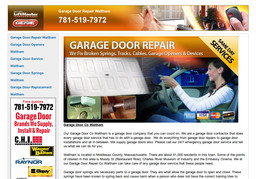In this image, we see a screenshot of a pixelated advertisement for a garage door repair service. At the top of the image, a phone number, 781-519-7972, is clearly displayed. Adjacent to this number are several pictures: the first depicts people pressing a button resembling a garage door remote control. Below this image, there's white text that reads "Garage Door Repair" with a smaller line of white text underneath it, which is difficult to decipher.

Further down, there are additional images illustrating various garage door-related activities: one shows a garage door opening, another portrays someone installing a component on the ceiling, and a third depicts an individual inside a car holding a garage remote. On the left side of the image, there is a column of blue text, with the phone number, 781-519-7972, displayed once more in black alongside the term "Garage Door." Beneath this, there is more red text which is largely indiscernible due to pixelation. Below the photos on the right side, several paragraphs of text appear in black on a white background, offering further details about the service, though the pixelation makes the content difficult to read.